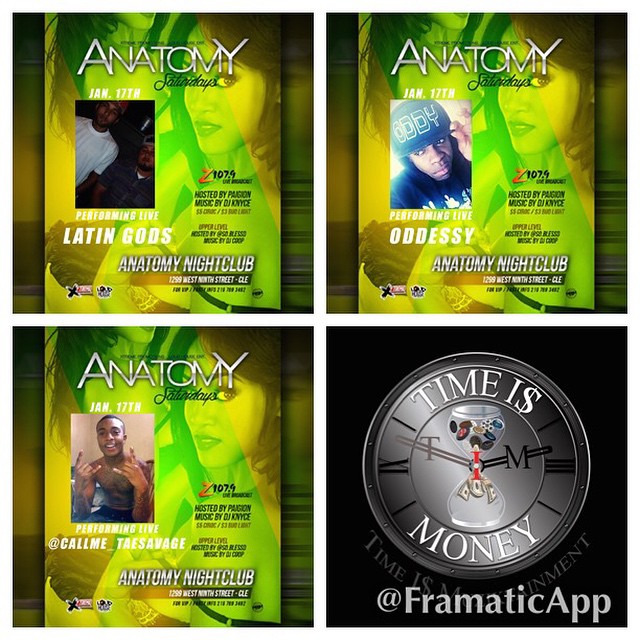The image is a square divided into four equal parts by a white cross, creating distinct top-left, top-right, bottom-left, and bottom-right sections. The top two images and the bottom-left image share a similar background: a green poster set against a copper-colored wall. The green poster features two images of the same woman, with the text "Anatomy Saturdays" in silver at the top and "Anatomy Nightclub" below. The dates on these posters are all January 17th. 

In the top-left section, a photograph of a person is labeled "Performing Live: Latin Gods." The top-right section has another photograph labeled "Performing Live: Odyssey." The bottom-left section features a third photograph labeled "Performing Live: Call Me T.A.E. Savage."

The bottom-right section of the image stands out with a black background. It features a silver clock design with an hourglass in the center. The hourglass has buttons at the top and dollar bills spilling out from the bottom. The words "Time Is" appear at the top in white print, with the 'S' stylized as a dollar sign, followed by the word “Money” underneath. The image is signed at the bottom with "@PhoneticApp."

Additionally, the top sections of the posters include details such as "Anatomy Saturdays Z107.9 Live Broadcast Hosted by Pygon, Music by DJ Night, Can Ice $5, Bud Light $3, Upper Level Hosted by @SoBlessed, Music by DJ Co-op, and Anatomy Nightclub 1299 West 9th Street CLE."